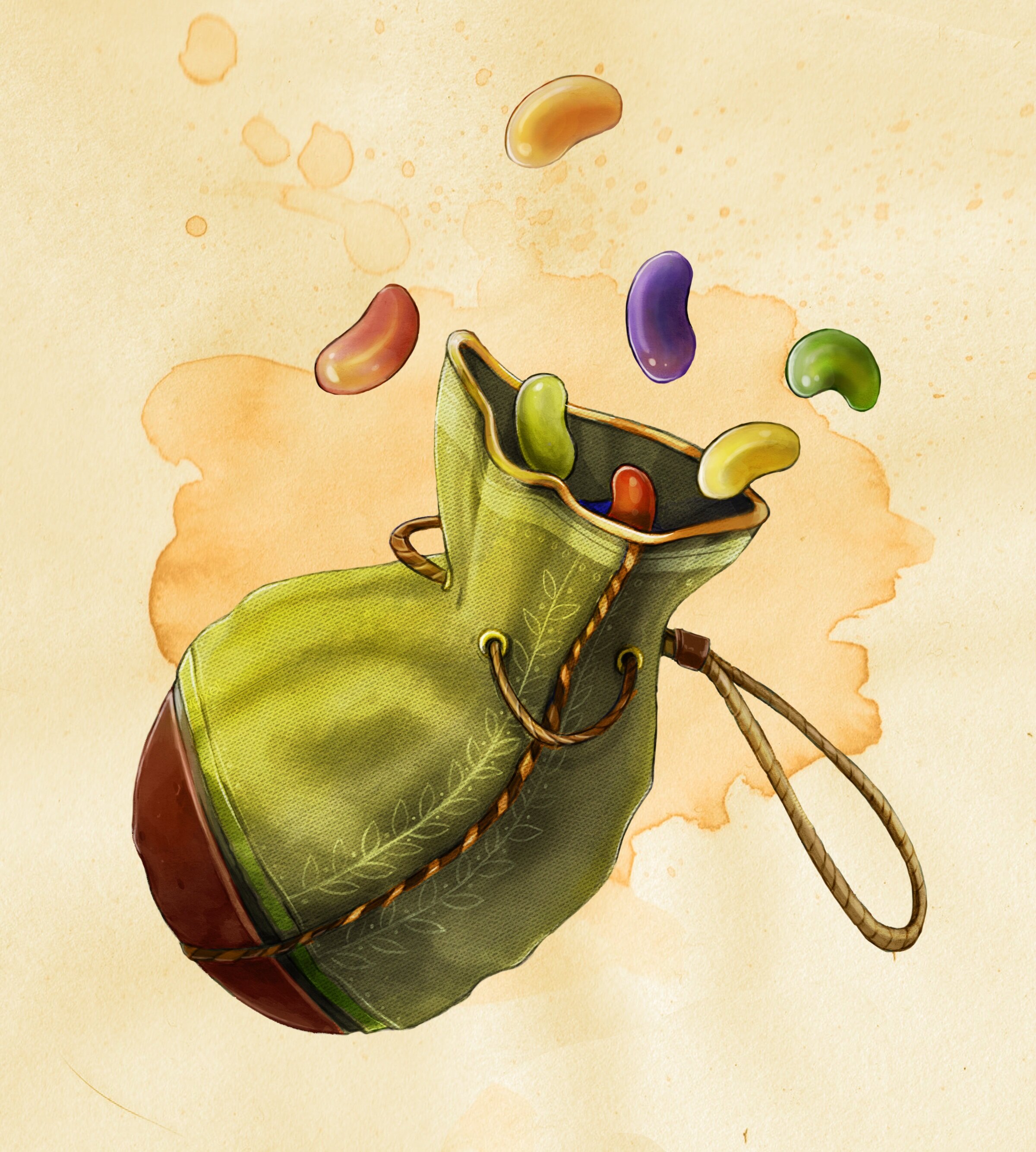This detailed watercolor illustration depicts a hand-crafted, green satchel with a brown leather base and a floral vine design running up the side alongside a drawstring. The satchel, cinched at the middle with a cord laced through eyelets, features a looped handle on the right side. It rests upon a light cream-colored background with a splotch resembling a pale brown ink stain at the center, accented by lighter dots above. Various colorful beans, resembling jelly beans in shades of red, yellow, purple, green, and orange, are spilling out of the top of the satchel and scatter over the watercolor splash below.